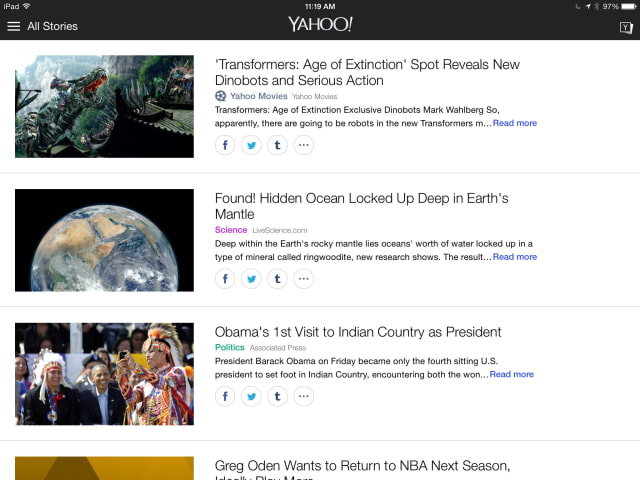This screenshot from an iPad displays the state of the device and an active session on Yahoo's website. The tablet is connected to a full Wi-Fi signal, with "Do Not Disturb" mode enabled and Bluetooth turned off. The battery is at 97%, and it is currently 11:19 a.m.

In the upper left corner, the word "iPad" confirms the device. The screen shows Yahoo's mobile site, identified by its distinctive logo and layout. In the top left, a hamburger menu icon provides access to various categories and stories. On the right, there's a "Y" in a square indicating additional menu options.

The page features several prominent news headlines with accompanying images. The primary article showcases a still from "Transformers: Age of Extinction," featuring new Dinobots, emphasizing intense action scenes. This exclusive content from Yahoo Movies highlights actors like Mark Wahlberg and encourages readers to delve deeper, offering sharing options across Facebook, Twitter, Tumblr, and more.

The second story discusses a scientific breakthrough, revealing a hidden ocean within Earth's mantle in minerals called ringwoodite. This piece from Live Science invites readers to explore new research findings, similarly supported by sharing possibilities.

Another headline focuses on President Barack Obama's historic visit to Indian country, documenting his interaction with Native Americans and marking him as only the fourth sitting U.S. president to do so. Although the excerpt trails off, it maintains an engaging tone, inviting further reading through provided links and sharing features.

Lastly, a partial headline indicates that Greg Oden is planning an NBA return next season, rounding out the snapshot of Yahoo's diverse news offerings. This detailed view underlines the breadth of stories available on Yahoo's iPad interface.